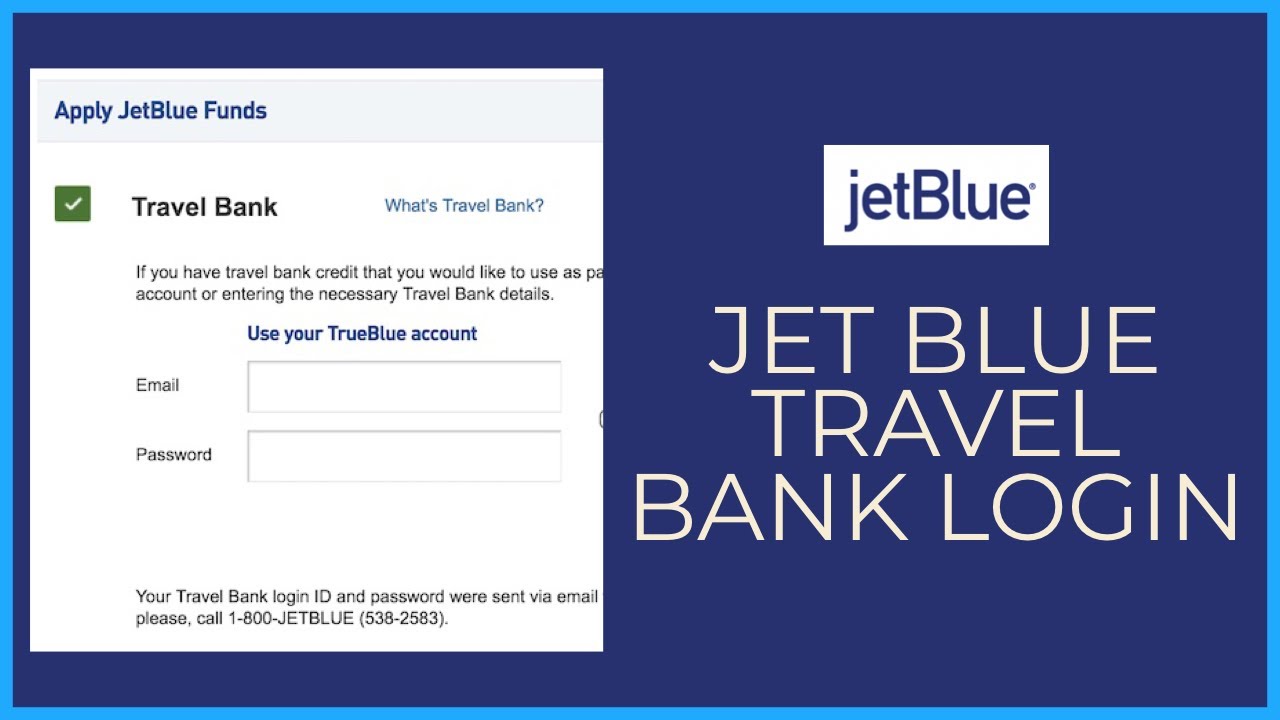The image depicts a rectangular interface for JetBlue's Travel Bank on a white background. At the top, there is a header with the JetBlue logo, with "Jet" in lowercase letters and "Blue" starting with an uppercase 'B', all in blue text within a white rectangle. Below the header, there is a checkbox labeled "Travel Bank" that is checked, accompanied by a blue hyperlink text that reads, "What’s Travel Bank?"

The caption then describes an instructional message that reads: "If you have Travel Bank credit that you would like to use as part of..." (with some words possibly cut off). On the next line, the text continues with: "...enter the necessary Travel Bank details."

Under this section, there are fields prompting for "Email" and "Password" alongside a blue button with the text, "Use your TrueBlue account." Near the bottom of the image, a text in blue states: "Your Travel Bank login ID and password, or sent via email, please call 1-800-JetBlue (538-2583)."

At the very bottom, there is another white rectangle featuring the words "JetBlue Travel Bank Login" in crisp blue text, aligned to guide users on how to access their Travel Bank funds. The overall interface appears to be user-friendly and geared towards JetBlue customers looking to manage their travel credits.